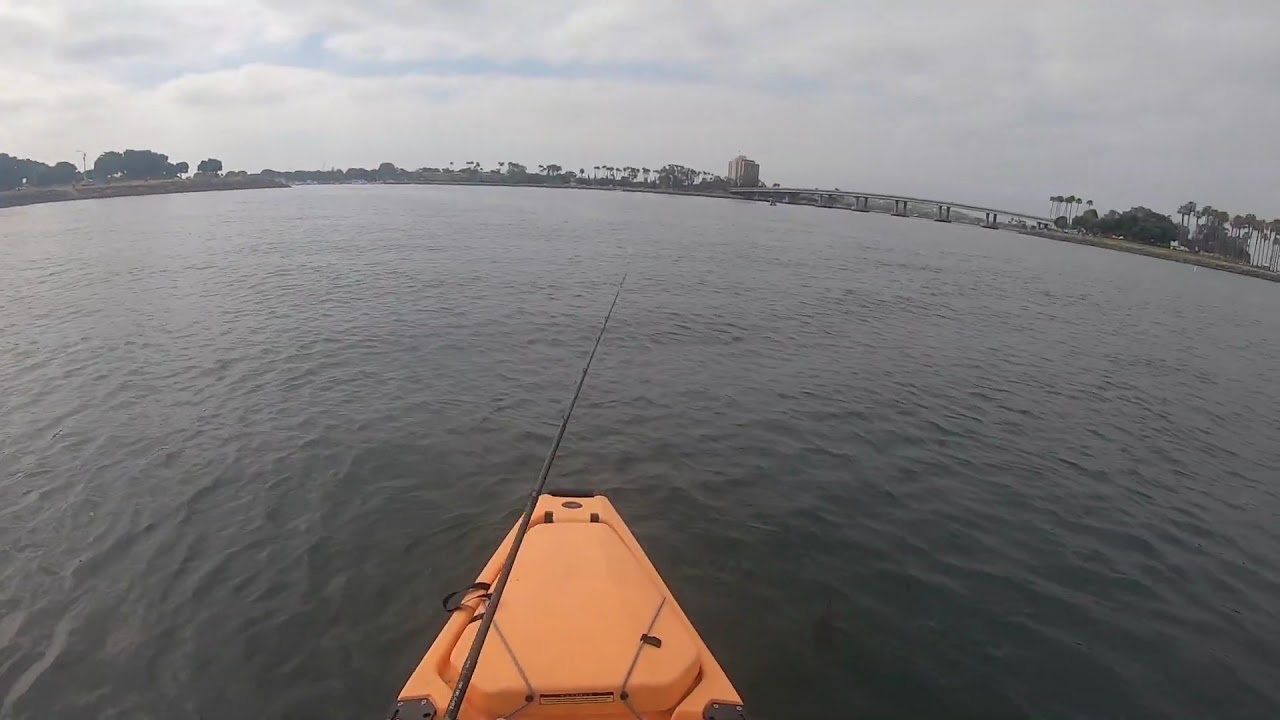This horizontally aligned rectangular image captures a serene kayaking experience from a first-person perspective. Dominating the foreground is the triangular front of an orange kayak, secured with red and gray rope, adding a touch of vivid color to the scene. Extending from the kayak towards the center of the image is a black fishing rod, hinting at a peaceful fishing adventure. The kayak is afloat on a dark blue body of water, which is gently rippled with small waves. Above, the sky is mostly gray with a mix of light and dark clouds, though patches of blue peek through. The horizon reveals a diverse shoreline: to the left is a dense array of green trees, to the right are tall palm trees, and in between stands a bridge connecting the two segments of land. Further into the background, a rectangular, multi-story building adds an element of urban contrast to the natural scenery. This image beautifully merges elements of tranquility and gentle motion, framed by both nature and human structures.